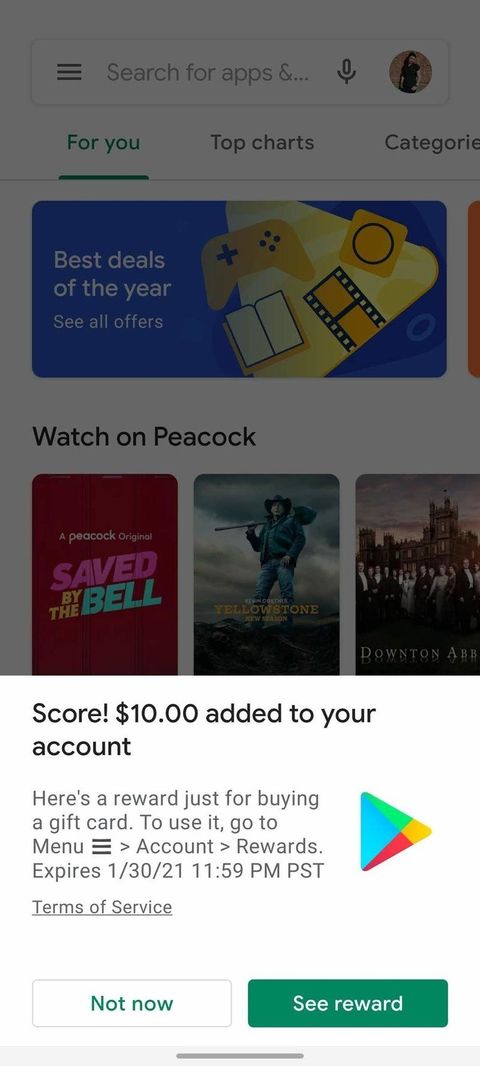A pop-up notification appears over a light gray background, highlighting a special reward. The pop-up itself has a white lower section and, in bold black text, it announces "SCORE!" followed by a message that $10.00 has been added to the user's account. The notification reads, "Here's a reward just for buying a gift card. To use it, go to the menu with the three lines, then select 'Account and Rewards'."

Important details include the expiration of the reward, which is listed as "10-30-21 at 11:59 PM PST." Below this, there's a smaller note directing users to review the "Terms of Service." 

At the bottom of the pop-up are two buttons: the first is white with green text saying "Not Now," and the second is green with white text stating "See Rewards." Alongside, there is a Google Play logo featuring the familiar blue, green, red, and yellow triangle.

Above the pop-up, the grayed-out background reveals further details. There's a search bar outlined in gray with placeholder text in gray reading, "Search for apps…" accompanied by a gray microphone icon. Adjacent to the search bar, there's a profile picture circle, showing a person in a black shirt.

Several tabs are visible beneath the search bar. The first tab labeled "For You" is green and underlined, indicating it is the current selection. Following tabs include "Top Charts" and "Categories" in gray text. Additionally, there is a blue rectangle promoting "Best Deals of the Year" with a "See All Features" link on the left. In black text, titles such as "Watch on Peacock," "Saved by the Bell," "Yellowstone," and a cut-off reference to "Downton Abbey" are mentioned.